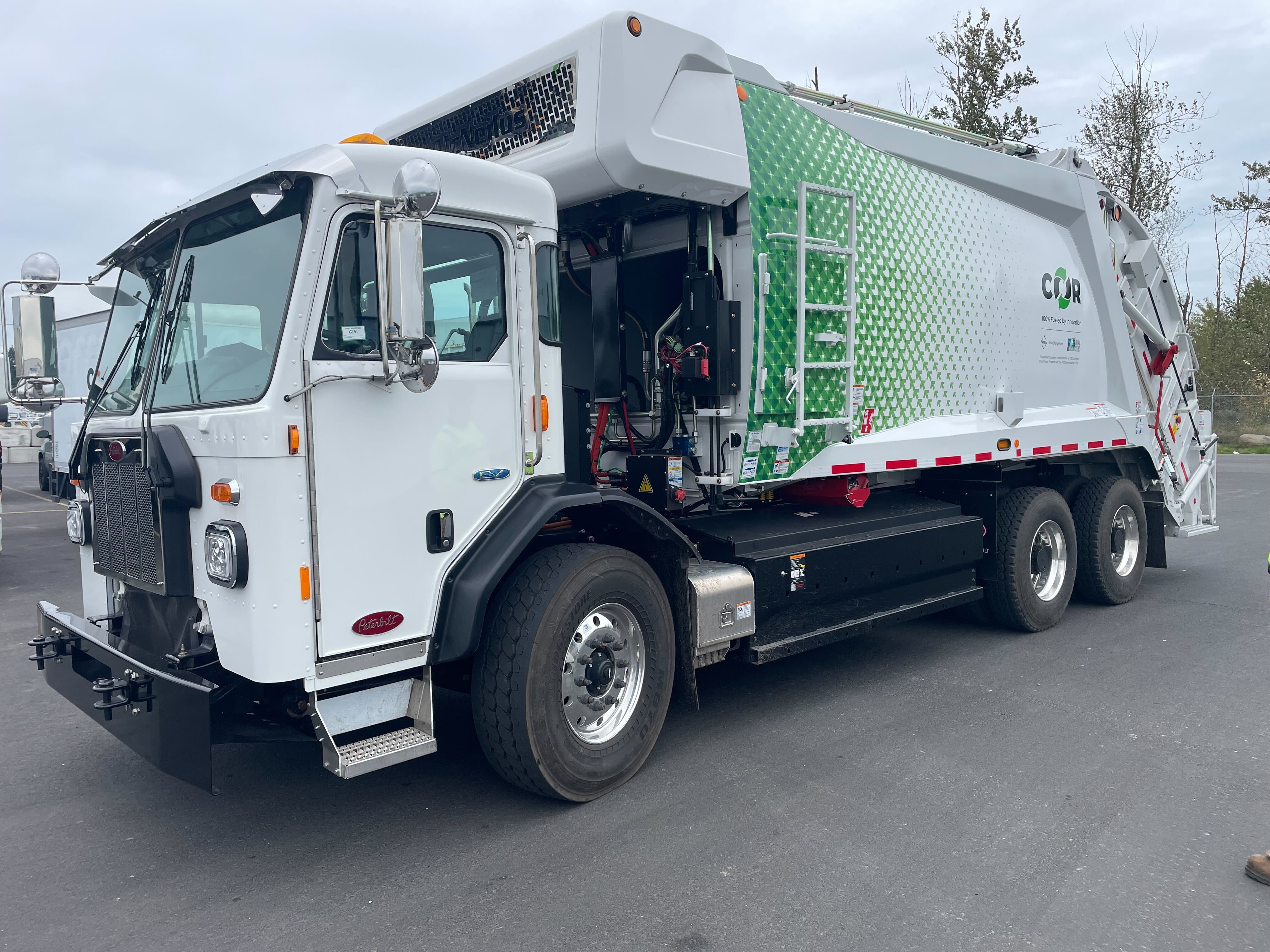The image depicts a realistic, horizontally oriented photograph taken during the day with a slightly overcast sky. A primarily white garbage truck, appearing almost new with a very large front window, dominates the scene. The truck is parked on what seems to be a clean, wide, asphalt parking lot. It is angled to the left, revealing its front left side and three visible wheels—one in the front and two at the rear, with possibly double rear wheels.

The front of the truck features a black bumper and a step up into the cab, while a large gas tank is noticeable on the driver's side. The truck's sides are adorned with a distinctive, scale-like green pattern that transitions from dark to lighter shades and incorporates increasing white spots as it descends. This pattern is overlaid by a white ladder. The truck’s rear displays a partially visible logo, appearing as "C-O-R".

In the background, on the left, industrial tanks can be seen, while sparse trees lie further out to the right. The setting and perspective give the photograph a slightly square feel, enhancing the detailed capture of the truck's features against the flat gray sky.